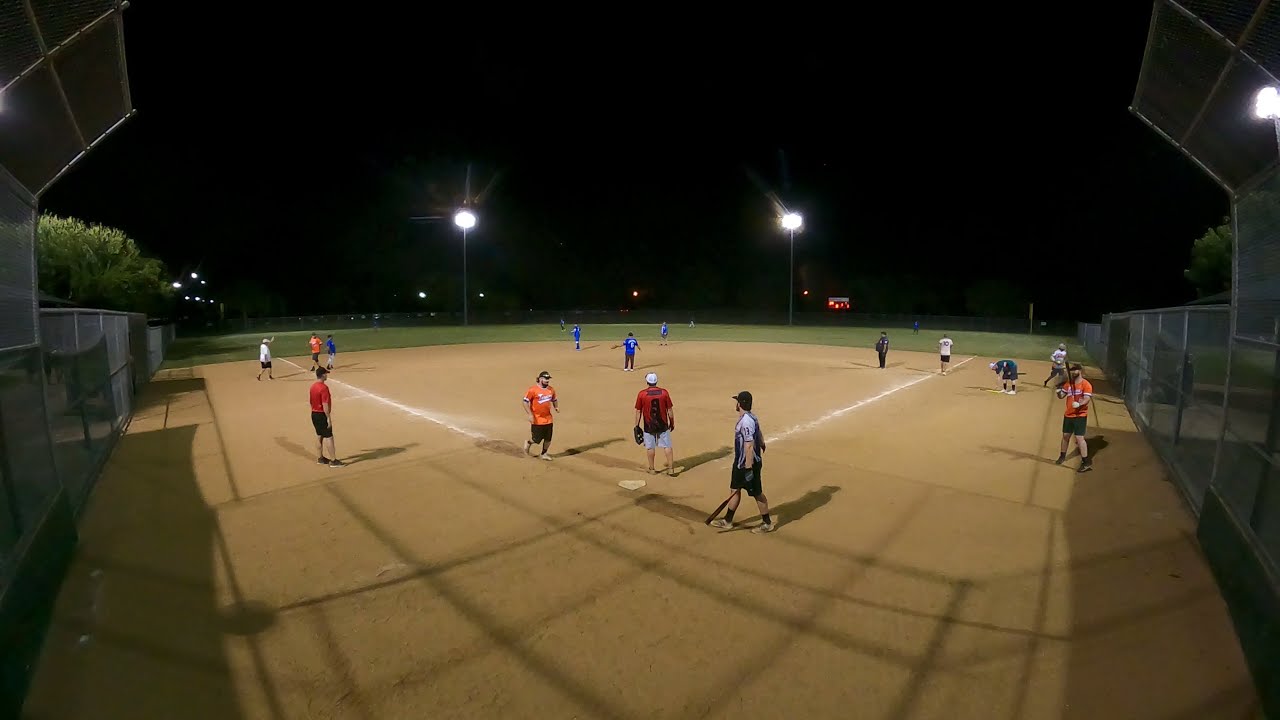This nighttime image captures a recreational baseball or softball game, most likely involving an older men's league. The sky is pitch black, illuminated by three sets of towering field lights positioned strategically around the green outfield. The field is enclosed by a chain-link fence, although it is unclear if the fence completely wraps around the outfield. From the vantage point behind home plate, the baseball diamond is clearly visible, with distinct chalk lines marking the baselines and dirt surrounding the bases.

On the field, a player in an orange shirt is seen jogging towards home plate. The defensive team, comprising at least the pitcher, shortstop, and second baseman, is clad in blue shirts. Additional players in the outfield also wear blue, while the team at bat has players wearing a mix of orange and possibly red.

Despite the active illumination, the scoreboard in the far background remains unreadable. The setup of the game, with no immediate hitter at the plate and players positioned in various roles, suggests a moment of transition in play. The protective cage around the home plate area is designed to prevent foul balls from reaching the spectators, indicating a thoughtful and safe playing environment.